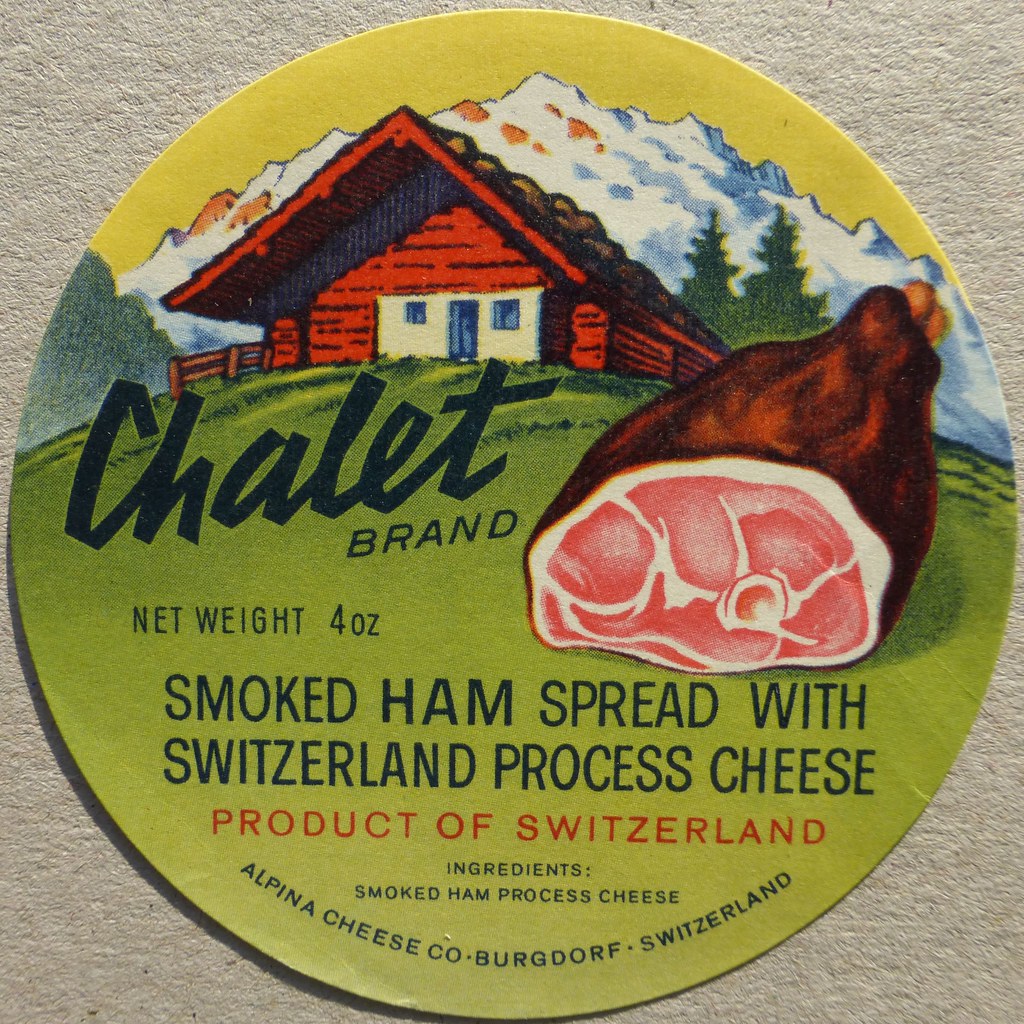This image features a square photograph of an old-style, circular food label set against a textured gray background that peeks through at the corners. The label is predominantly green and includes a vibrant illustration of a scenic Switzerland countryside. At the top, there's a wooden cabin nestled atop a green hill with snow-capped mountains behind it, framed by pine trees. Above this picturesque setting, a yellow sky suggests a sunlit background.

Central to the label is the brand name "Chalet" prominently displayed in large cursive black letters, followed by the word "brand" in smaller print. To the right of the text, an illustration of a smoked ham, pink with a brown exterior and a visible bone, captures attention. Below the name, the label reads in bold black uppercase letters: "smoked ham spread with Switzerland processed cheese," with "net weight 4 ounces" positioned above this description. An orange caption beneath announces "Product of Switzerland."

Further details include a list of ingredients—smoked ham and processed cheese—and the label indicates it is a product of the Alpina Cheese Company, Bergdorf, Switzerland. The overall colorful and detailed artwork reflects a quaint, rural Swiss ambiance, indicative of the ham spread with cheese that it advertises, likely intended for use on crackers or similar snacks.